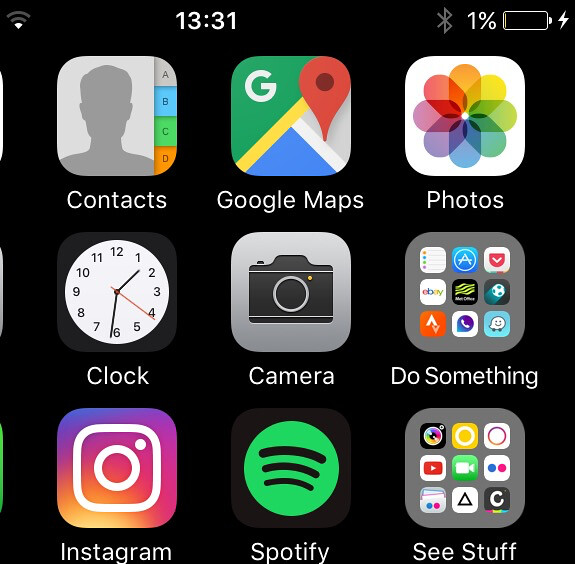The image appears to be a screenshot of a smartphone home screen. The layout is a grid of app icons arranged in a 3x3 square pattern. Here’s a detailed breakdown:

- **Top Bar:**
  - The status bar shows the time as 13:31.
  - It includes an unilluminated Wi-Fi icon, indicating no active Wi-Fi connection.
  - The battery icon displays a critical charge of just 1%.

- **App Icons:**
  - **Top Row (from left to right):**
    - **Contacts Icon**
    - **Google Maps Icon**
    - **Photos Icon**

  - **Second Row:**
    - **Clock Icon**
    - **Camera Icon**
    - **A folder labeled "Do Something" containing various app icons:**
      - eBay
      - A note-taking app
      - Possibly a sports channel app

  - **Third Row:**
    - **Instagram Icon**
    - **Spotify Icon**
    - **Another folder labeled "See Stuff" containing app icons:**
      - Various unidentified apps

- **Bottom Collection (3x3 arrangement):**
  - **Top Row:**
    - **Camera App Icon**
    - **An app possibly for Oros Ring**
    - **YouTube Icon**

  - **Second Row:**
    - **Video Camera Icon**
    - **A Triangle Icon**
    - **An icon with the letter "C"**

- **Other Details:**
  - The black background provides a sleek contrast to the colorful app icons.
  - The clock widget at the bottom also shows 13:31.

This detailed menu layout showcases a variety of commonly used applications and folders on a mobile device with a minimalistic black theme.